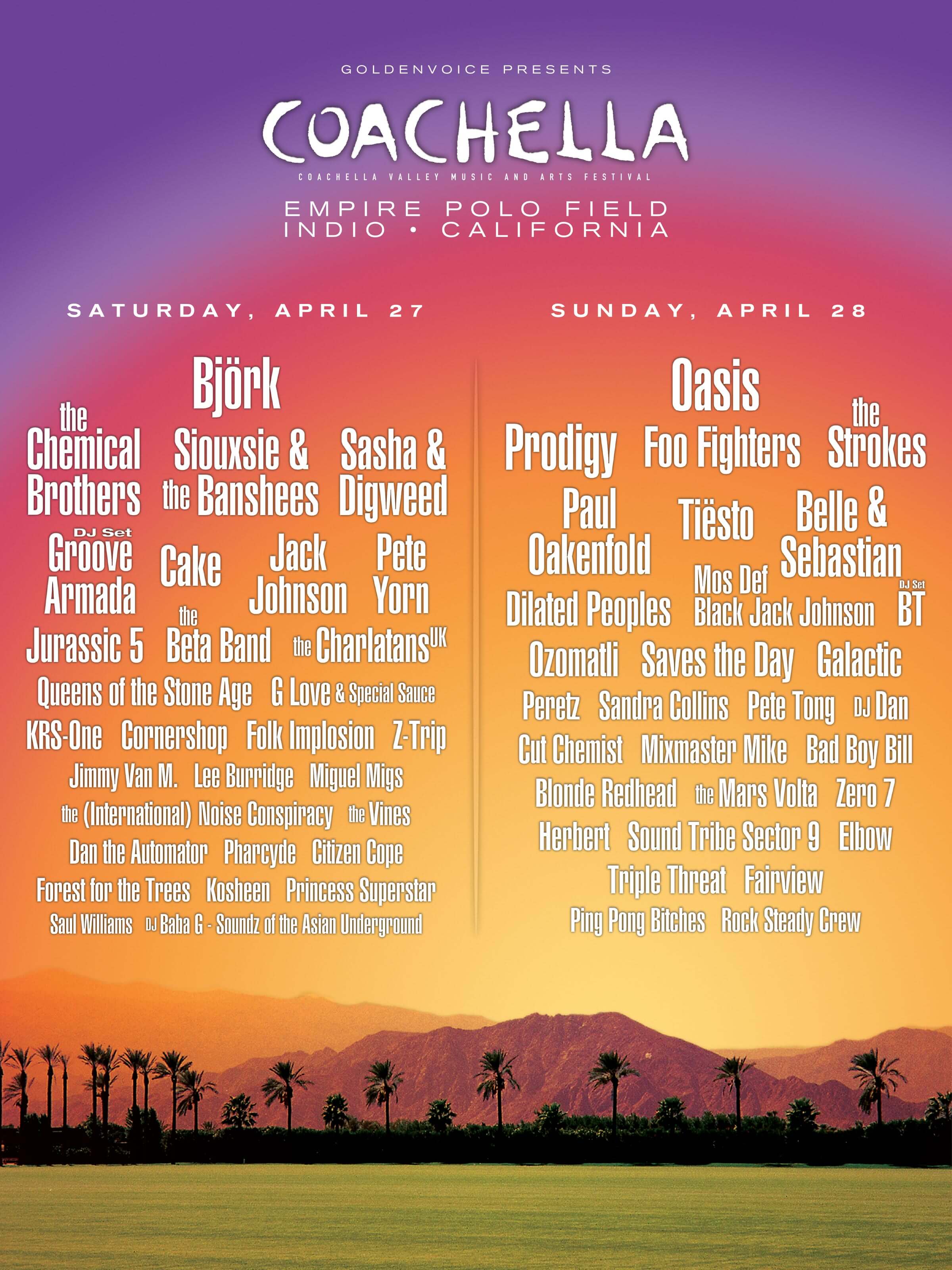The colorful Coachella poster features a vibrant sky in shades of yellow, orange, pink, and purple, with a green grass field, palm trees, and a distant mountain range. The top of the poster reads "Golden Voice presents Coachella Valley Music and Arts Festival" in white lettering. Located at the Empire Polo Field in Indio, California, the festival is split into two days: Saturday, April 27th, and Sunday, April 28th. The lineup includes a mix of renowned and diverse artists. Saturday's headliners are Bjork, The Chemical Brothers, Suzy and the Banshees, Sasha and Digweed, Groove Armada, Cake, Jack Johnson, Pete Yorn, Jurassic 5, The Beta Band, The Charlatans UK, Queens of the Stone Age, G Love and Special Sauce, KRS-One, Cornershop, Folk Explosion, Z-Trip, Jimmy Van M, Lee Burridge, Miguel Migs, The International Noise Conspiracy, The Vines, Dan the Automator, Paracycle, Citizen Cope, Forest for the Trees, Cochine, Princess Superstar, Saul Williams, DJ Baba G, and Sounds of the Asian Underground. Sunday's lineup features Oasis, Prodigy, Foo Fighters, The Strokes, Paul Oakenfold, Tiesto, Belle and Sebastian, Dilated Peoples, Mos Def, Black Jack Johnson, DJ BT, Amomati, Saves the Day, Galactic, Sandra Collins, Pete Tong, DJ Jan, Cut Chemist, Max, Mister Mike, Bad Boy Bill, Blonde Redhead, The Mars Volta, Zero 7, Herbert, Sound Tribe Sector 9, Elbow, Triple Threat, Prefuse 73, Ping-Pong Bitches, and Rock Steady Crew. The poster's text becomes increasingly smaller towards the bottom, listing the extensive lineup of artists for the event.